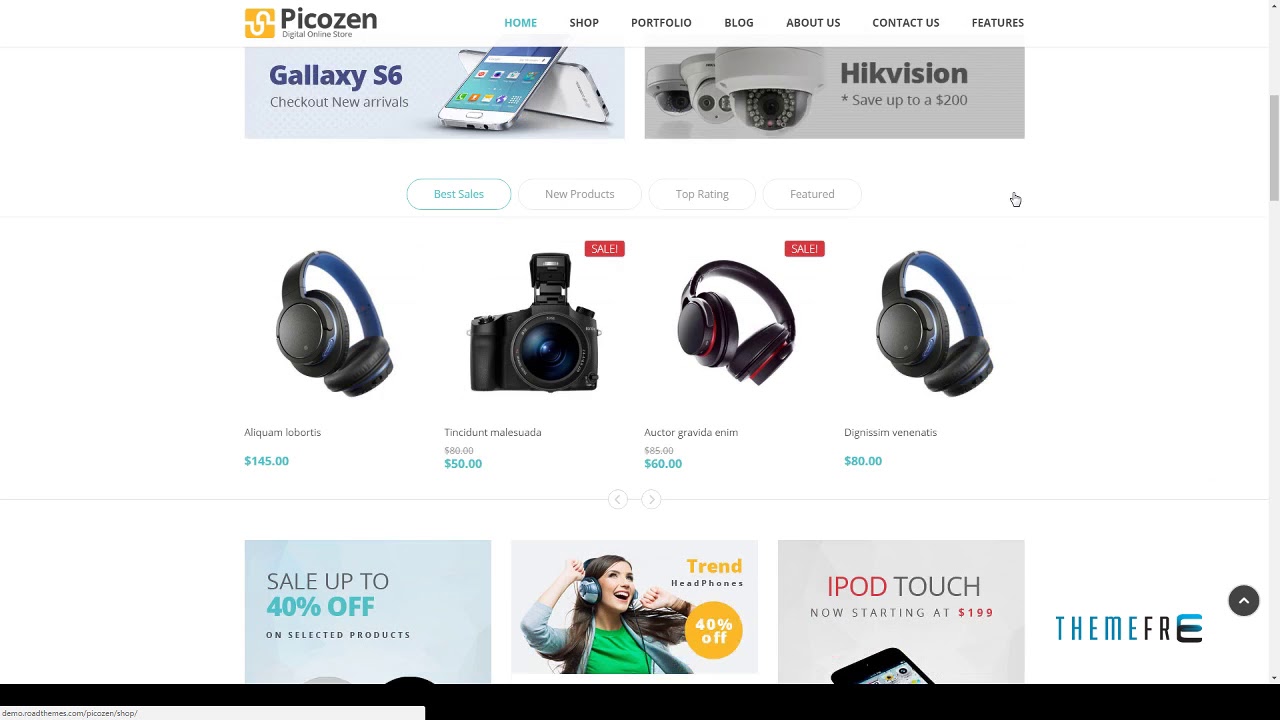Screenshot Description:

The screenshot displays a section of Pico's online store showcasing various features and products. The navigation menu at the top includes tabs for "Home," "Shop," "Portfolio," "Blog," "About Us," "Contact Us," and "Features," with the "Home" tab highlighted in blue. The main promotion on the page highlights the "Galaxy S6," and prompts visitors to "Check Out New Arrivals," emphasizing two phone models. 

A featured banner titled "PeakVision" announces a savings offer of "up to $200" (noted with an asterisk). Below, a "Best Sales" section is highlighted in blue, showcasing new products at the top in a tab format. 

Four product images are displayed in this section:
1. A pair of blue headphones priced at $145.
2. A camera priced at $50.
3. Another pair of red headphones priced at $60.
4. A pair of blue headphones priced at $80.

At the bottom of the screenshot are promotional banners, including one offering "Up to 40% off on selected products." Another highlighted promotion features a picture of a girl wearing headphones, with the text "Trend Headphones - 40% off" written in white and enclosed in a yellow circle.